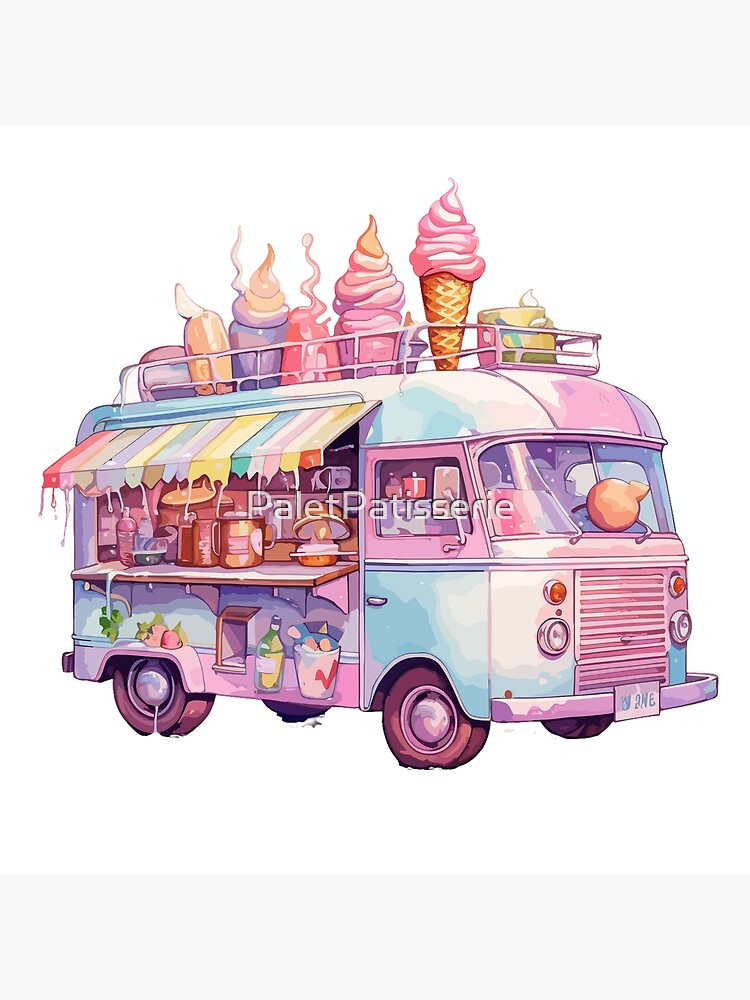This vibrant watercolor and pastel illustration depicts a whimsical ice cream or dessert food truck, modeled after a vintage Volkswagen bus. The truck is adorned in an array of pastel hues, including blue, white, pink, magenta, yellow, and green, creating a splotchy, colorful appearance. The name "P-A-L-E-T Patisserie" is emblazoned on the side, hinting at an artisanal touch. A rainbow-striped awning extends over the serving area, offering a welcoming, festive vibe with its yellow, green, pink, and red stripes. Underneath, the side panel is decorated with playful images of bottles, fruits, and a bucket. Atop the vehicle, secured by a metal rack, are five oversized, vividly colored ice cream cones, purely decorative and adding to the truck's charm.